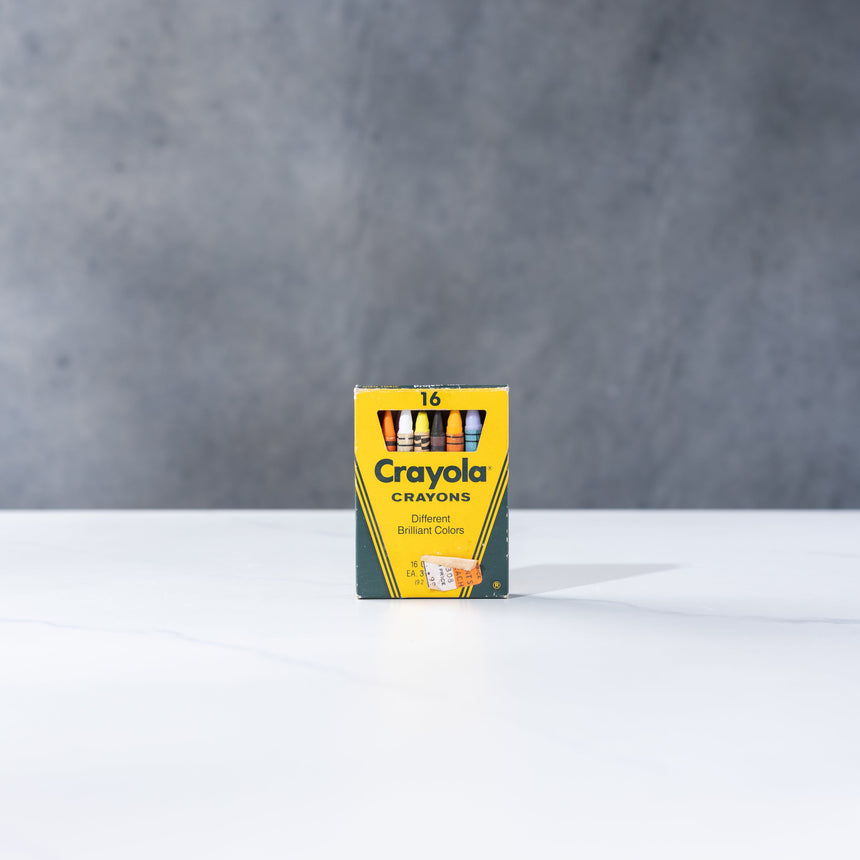The photo captures a vintage yellow Crayola box of 16 crayons, sitting on a white surface against a gray background. The well-worn box features dark green lettering for "Crayola" at the upper middle part of the package, with the words "Crayons" in bold dark green letters below it and “different brilliant colors” in slightly less bold green lettering at the bottom. The edges of the box are noticeably rubbed white, indicating its age. It displays vibrant crayons visible through a small front window, showcasing the colors orange, white, yellow, purple, yellow-orange, and a lighter blue. The box has green accents at the bottom corners and striping, with a partially peeled white and orange price tag towards the bottom right, adding to its retro charm from possibly the 1980s.